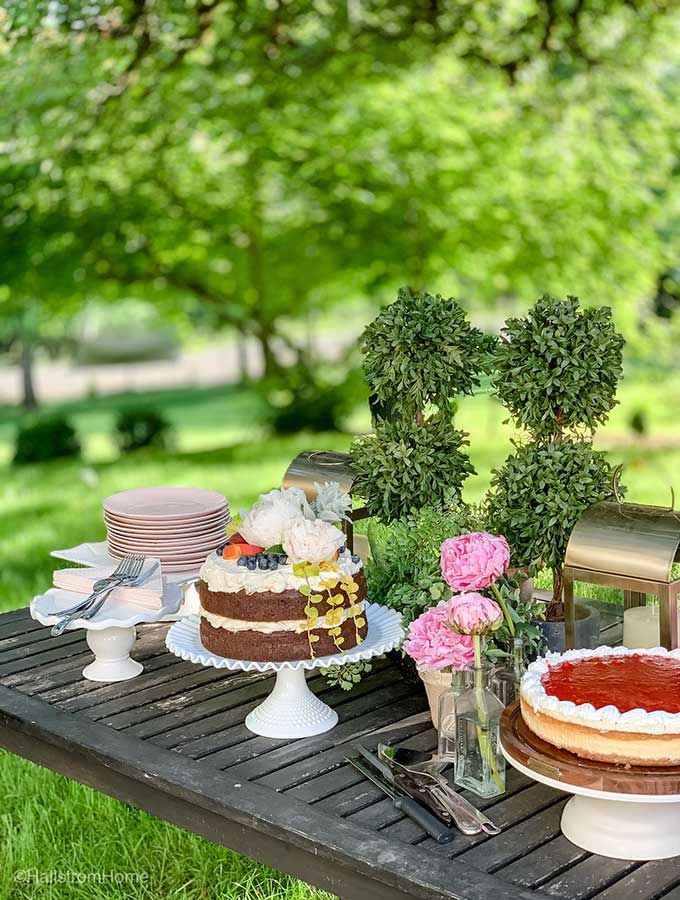The image showcases a serene outdoor setting featuring a rustic, gray wooden picnic table marked with scuffs and character. The table, bathed in natural light under a lush canopy of overarching trees and surrounded by verdant grass, is elegantly set as if for a leisurely garden gathering. Central to the display is an array of delectable desserts: a double chocolate layer cake adorned with blueberries and floral decorations, and a cheesecake topped with a red fruit jelly and bordered by white frosting. Both cakes sit invitingly on white frilly cake stands. Additionally, the table holds a collection of serving utensils, including forks, knives, and cake cutters, neatly arranged alongside stacks of plates and napkins.

The display is further complemented by decorative elements such as brass candle holders with candles, adding a touch of elegance, and vibrant, pink flowers arranged in a small jar and a clear glass vase, likely romunculuses. Small bonsai plants and a striking green foliage-shaped plant enhance the natural ambiance. Tucked towards the back are two metal chafing dishes with lids, hinting at a more extensive spread of offerings. Though a watermark is visible in the lower left corner of the image, the text remains indistinct, reading something like "home." The overall scene exudes calm and beauty, inviting viewers to imagine themselves partaking in this charming outdoor feast.